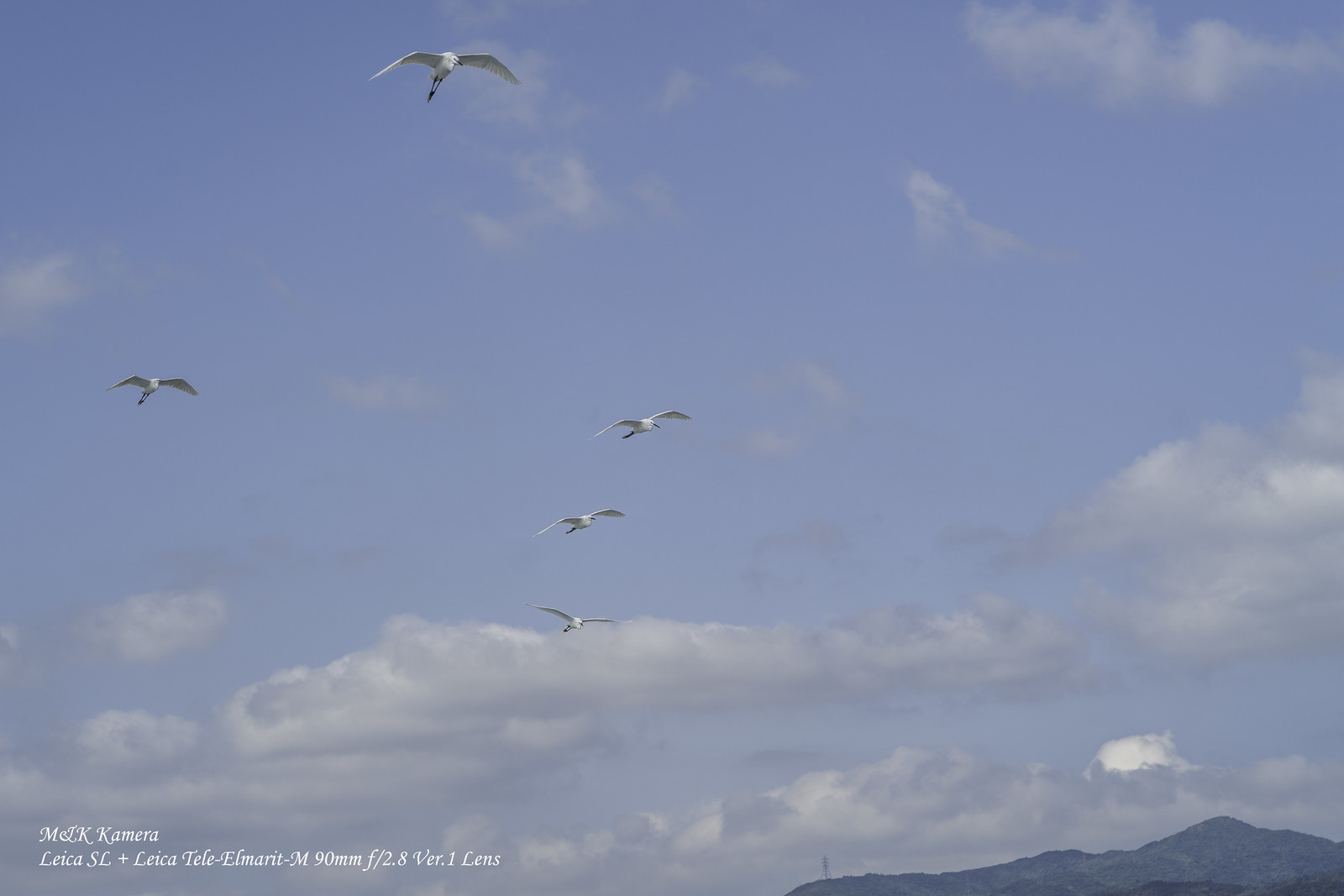This captivating photograph, taken by Mel K. Camera with a Leica SL and a Leica Tele-Elmarit M 90mm f/2.8 Version 1 lens, captures a tranquil blue sky adorned with scattered white, puffy clouds and hints of forming storm clouds. From a ground-up perspective, the image showcases five seagulls gracefully gliding towards the right. The birds, depicted from their underside, display their white bodies with distinct M-shaped wing formations, some seemingly coasting on the air currents. These seagulls, positioned in various spots across the sky, navigate towards a distant mountain, which has a bluish hue. The image is punctuated by text in the bottom left corner, which reads "Milk Camera, Lely SC, Lela, Tele Element, M, 90mm, 2.8, Version 1, Scent Lens."